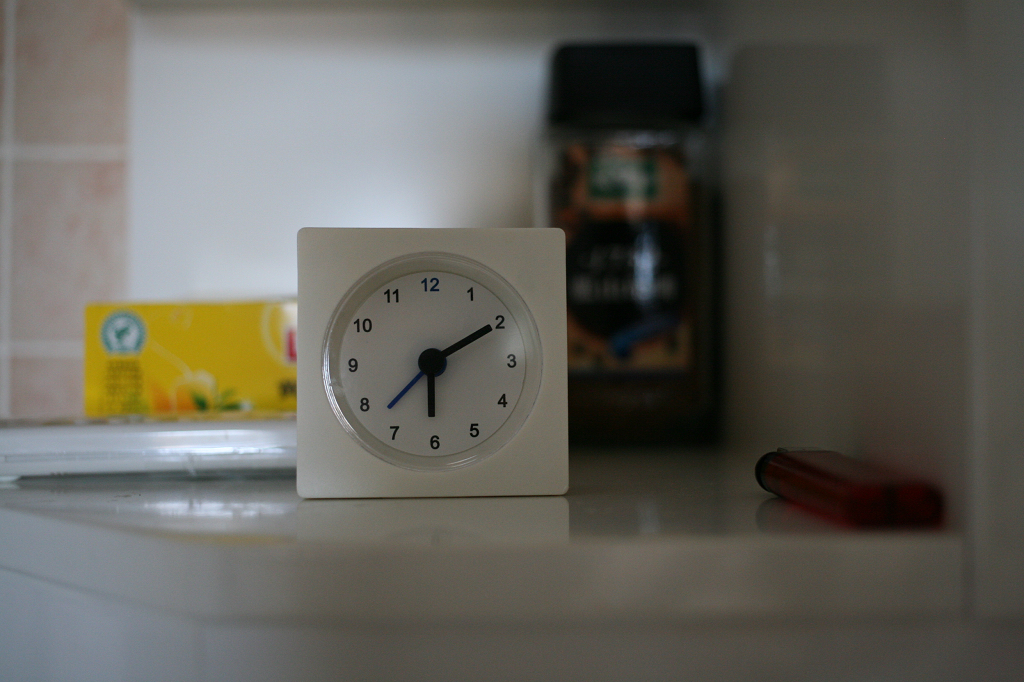The image features a small, square, white clock prominently positioned on top of a white shelf, which is part of what looks like a kitchen counter area with white cabinets underneath. The clock, which is the main focal point of the image, has a clear white face with black numbers ranging from 1 to 12. The clock hands indicate the time as 6:10, with the small hand on the six and the big hand on the two, and the second hand appears to be at around the 37-second mark. Behind the clock is a yellow box with multiple labels in blue, red, green, and white, depicting plants with orange flowers and green leaves. A dark brown glass jar, likely an instant coffee container with labels in green, yellow, and red, sits nearby. On the right side of the image is a clear plastic bottle with a black label and black lid. There's a red lighter lying on the white counter at the bottom right corner. The background includes a wall with peach and white tiles on the left side transitioning to an all-white portion. The overall image is somewhat blurry except for the well-focused clock in the center.